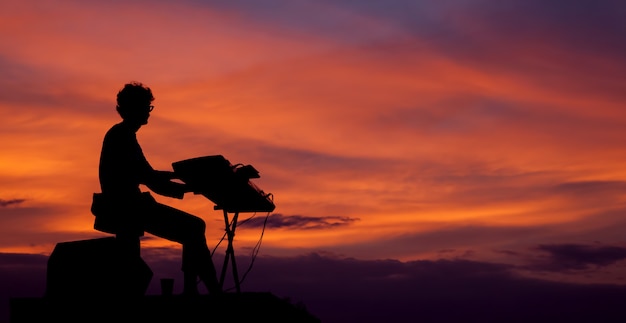The photograph depicts a silhouette of a person, likely a man with short, curly or wavy hair and glasses, seated at a keyboard. He is positioned towards the left side of this landscape-oriented image. The silhouette sits on a chair, with an object resembling an amplifier below him, connected by wires to the keyboard. The scene is set against a stunning sunset backdrop, characterized by dark orangish, purplish, and greyish streaked clouds that give the impression he is playing amidst the sky. The lighting and shading strongly suggest this is a sunset rather than a sunrise, enveloping the scene in a mystical and serene twilight atmosphere.